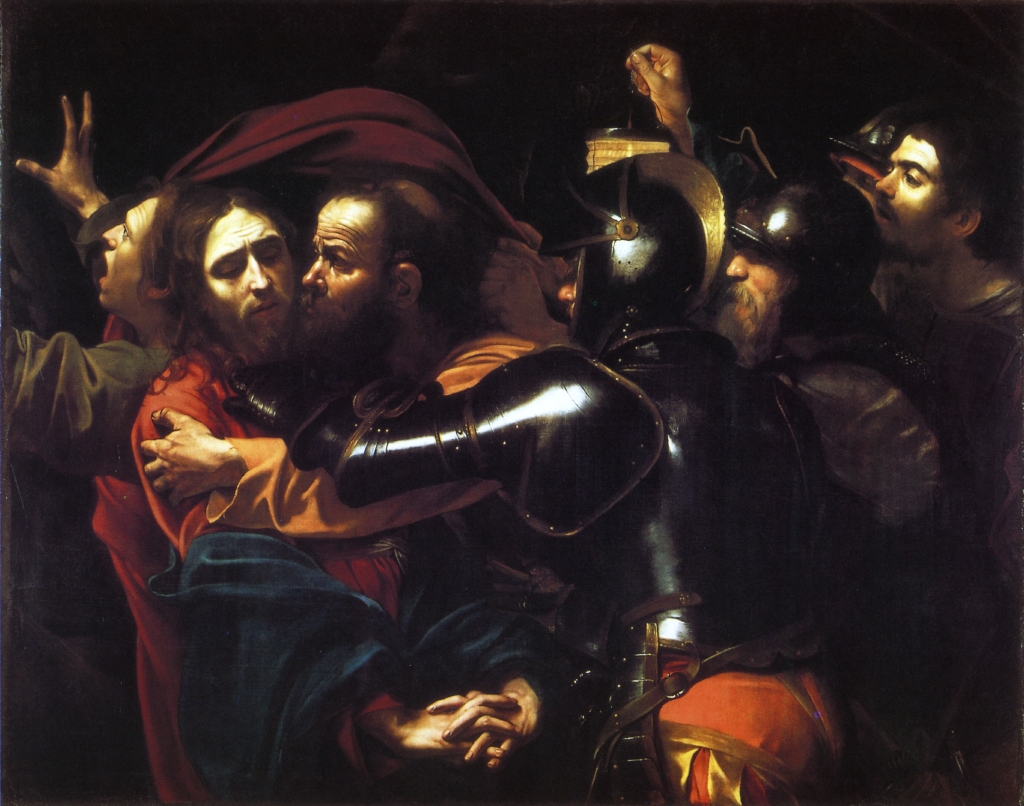In this detailed painting reminiscent of Michelangelo's work, a dramatic scene unfolds with several men, some dressed in black armor and others in vibrant robes. Central to the composition are two men in an emotional embrace, their fingers intertwined, suggesting fear or sorrow. One of these men, who closely resembles Jesus with his long brown hair and beard, is being held by another robed figure who has a bald patch at the back of his head. Surrounding them is a chaotic assembly of soldiers and onlookers.

A man in dark, shiny armor appears to be forcefully detaining the pair, his black hood partially obscuring his stern face. Behind him, another armored figure with a white beard watches intently, his expression illuminated by a lamp held by a man positioned further back. This lamp casts a golden light, contrasting with the dark and somber colors of the soldiers' armor. On the far left, a man with an anguished expression raises his hands to the sky, mouth open as if shouting, adding to the scene's tension and urgency.

The vivid detailing in the clothing and the interplay of light and shadow contribute to the painting's striking portrayal of a moment fraught with emotion and conflict, possibly depicting a historical or biblical event. The array of colors in the robes—orange, blue, red, and green—alongside the metallic sheen of the armor, creates a visually rich tapestry that draws the viewer into its story of struggle and confrontation.